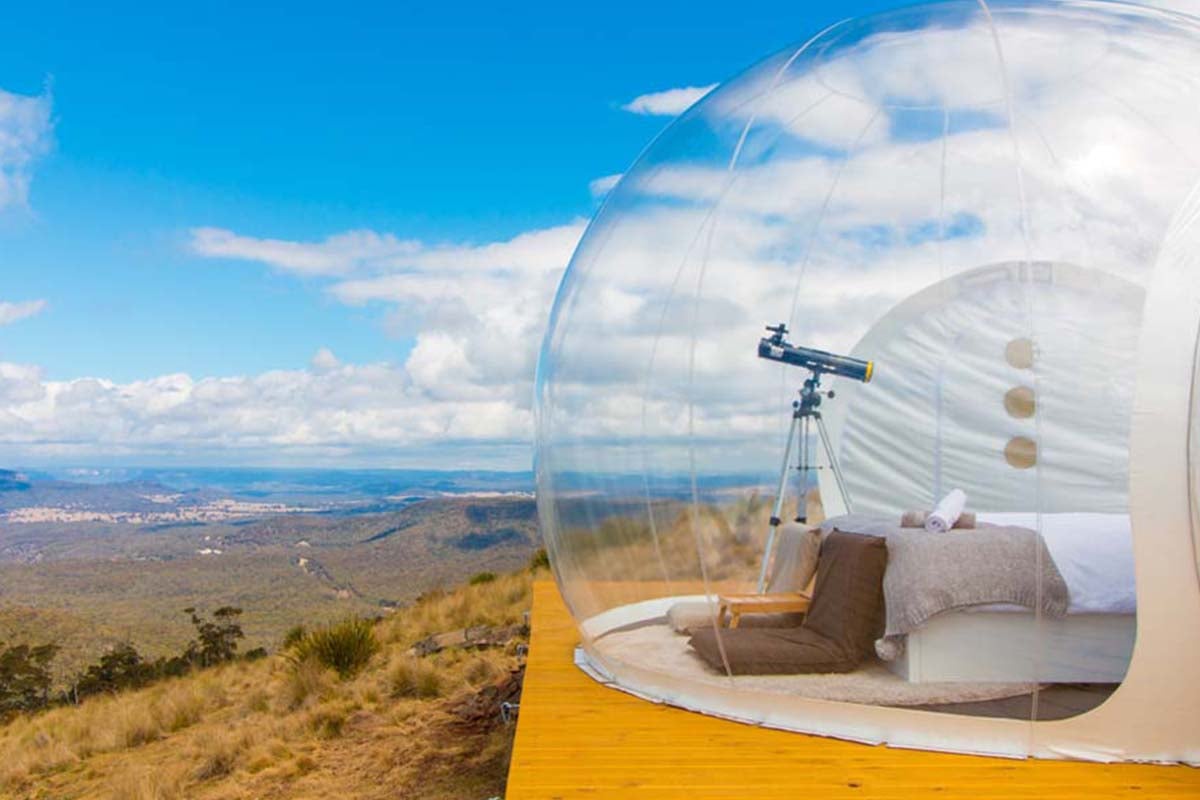The photograph captures an unusual, captivating scene set in the vast, dry landscape of what appears to be Arizona, on a clear, sunny day. On the right side of the image sits a wooden platform, atop which is a large, transparent, dome-shaped bubble tent. Within this clear bubble, a cozy interior is visible, featuring a made bed with white sheets and a tan blanket, a small table, two floor cushions—one dark brown and one light brown—and most notably, a telescope positioned for stargazing or observing the expansive surroundings. Adjacent to it, there's another similar bubble tent. The landscape extends into relatively flat terrain with sporadic hills and dry grass, a few trees, and a predominantly brown coloration, suggesting arid conditions. In the backdrop, the scenery blends into the horizon marked by rolling mountains and a bright blue sky dotted with fluffy white clouds.